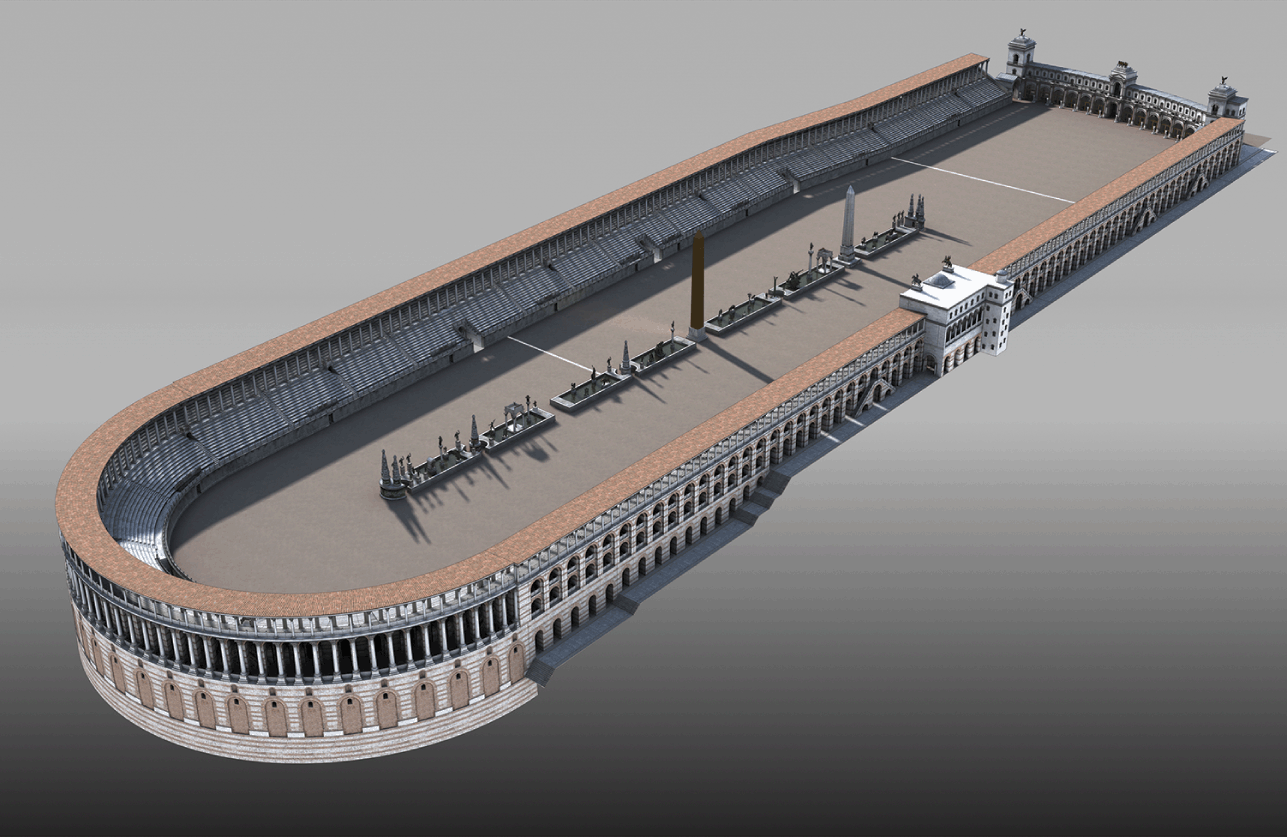In this highly detailed and realistic illustration, set against a background that transitions from light gray to a deep brownish-black, there is a central structure resembling an ancient walled stadium or coliseum. The walled area, resembling an elongated U-shape, is composed of concrete with oval-shaped openings at its base. This horseshoe-shaped enclosure features a majestic entranceway akin to medieval castle gates at the upper right corner. Surrounding the structure, a series of windows line the upper portions, while a series of paddle-like objects are seen at the bottom.

Inside the U-shaped structure, in the central courtyard, there are three groups of rectangular platforms. These platforms are adorned with indistinct, blurry objects that could be statues or fountains, adding an enigmatic feel to the scene. While the illustration is not immediately clear as to whether it depicts a modern or historical context, it effectively conjures the image of a significant architectural landmark, perhaps used for public gatherings or events, blending elements from both realistic art and historical architecture.